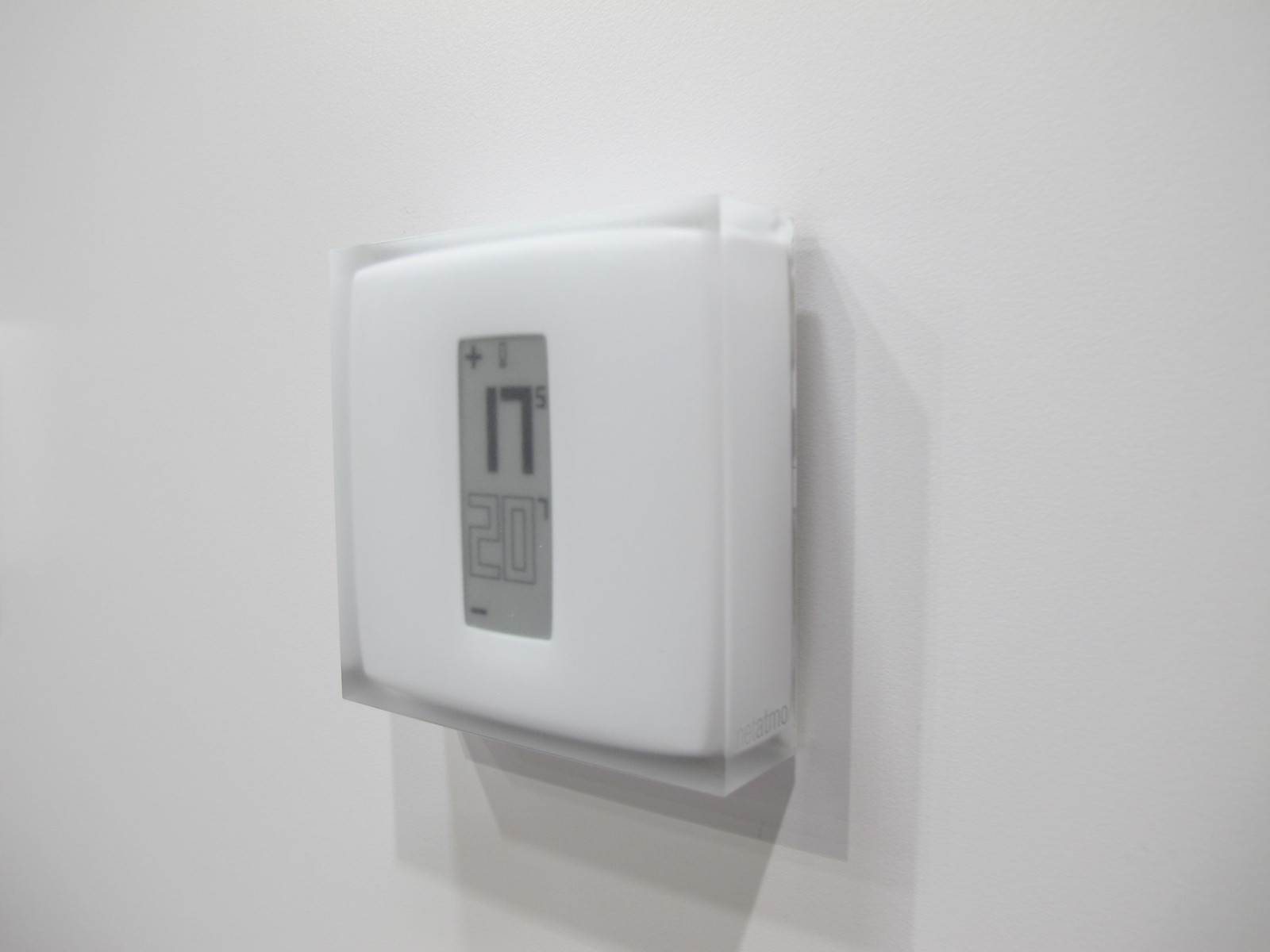The image prominently features a minimalist thermostat centered against a plain white wall. The thermostat itself is a sleek, white square design with a subtle, thin clear border around it, emphasizing its modern, simplistic aesthetic. At the forefront of the device is an electronic display, featuring the large number "17" in the center, likely indicating the current temperature setting. In the top right corner of the display, the number "5" is visible, perhaps representing a different setting or mode. Above the main display area, there is a plus (+) sign, indicating an option to increase the temperature, while at the bottom of the display, a black-outlined "20" is present alongside a minus (-) sign, presumably for lowering the temperature. The exact temperature unit (Celsius or Fahrenheit) is not specified. There are no other visible controls or features on the thermostat, and the rest of the shot maintains a clean, uncluttered look with the blank white wall accentuating the focus on the thermostat.